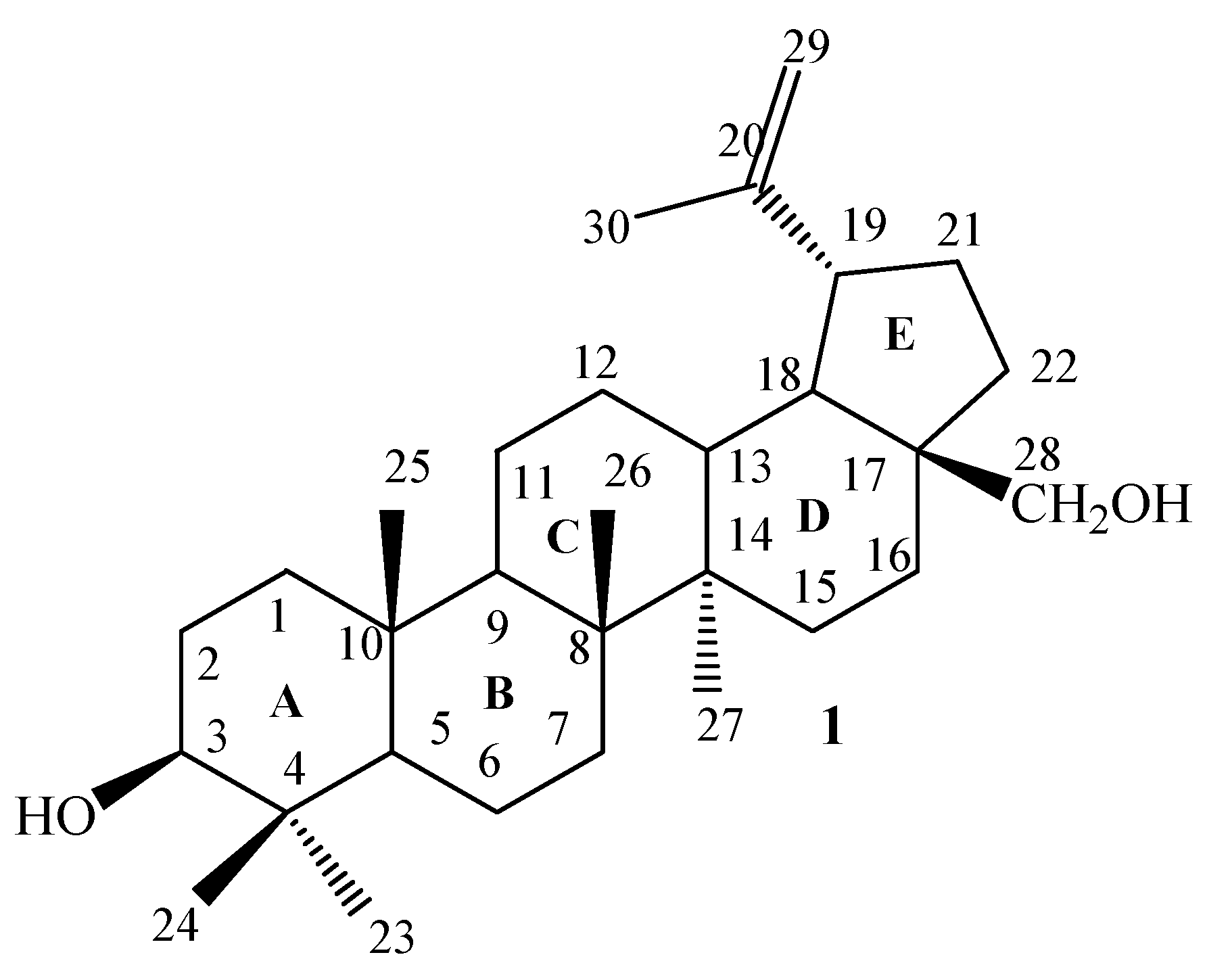The image displays a detailed black-and-white molecular diagram central to organic chemistry, illustrating a complex chemical structure composed of interconnected benzene rings and other shapes with various attached atoms and groups. 

Starting from the lower-left, there is a hexagon labeled 'A' with numbered carbon atoms at its vertices from 1 to 4 and 10. This ring has an HO (hydroxyl) group pointing to the third carbon. Adjacent to it, the image continues with a sequential numbering of carbon atoms, represented in a connected hexagonal ring labeled 'B.' The rings are interconnected, continuing this pattern with labels and numbers: the B ring extends the sequence through carbons 5 to 9 and includes external numbers like 25 and 26 positioned at the top and bottom, respectively.

The next hexagon, labeled 'C,' joins at carbon 11, covers carbons 11 to 16, and includes an external CH2OH group connected at carbon 17. Further along, the structure branches into a pentagon labeled 'E,' continuing the carbon numbering from 18 to 22, with important group attachments like a double bond between carbons 29 and 20. Additional notations include downward arrows and sonic wave-like patterns indicating positions and directions of particular bonds and groups.

Overall, the diagram intricately details the molecular architecture with interconnected hexagonal and pentagonal rings, systematically numbered carbon atoms, and diverse attachments, making it an illustrative example for those versed in organic chemistry. This comprehensive depiction aids in understanding the molecular structure's complexity and connectivity.